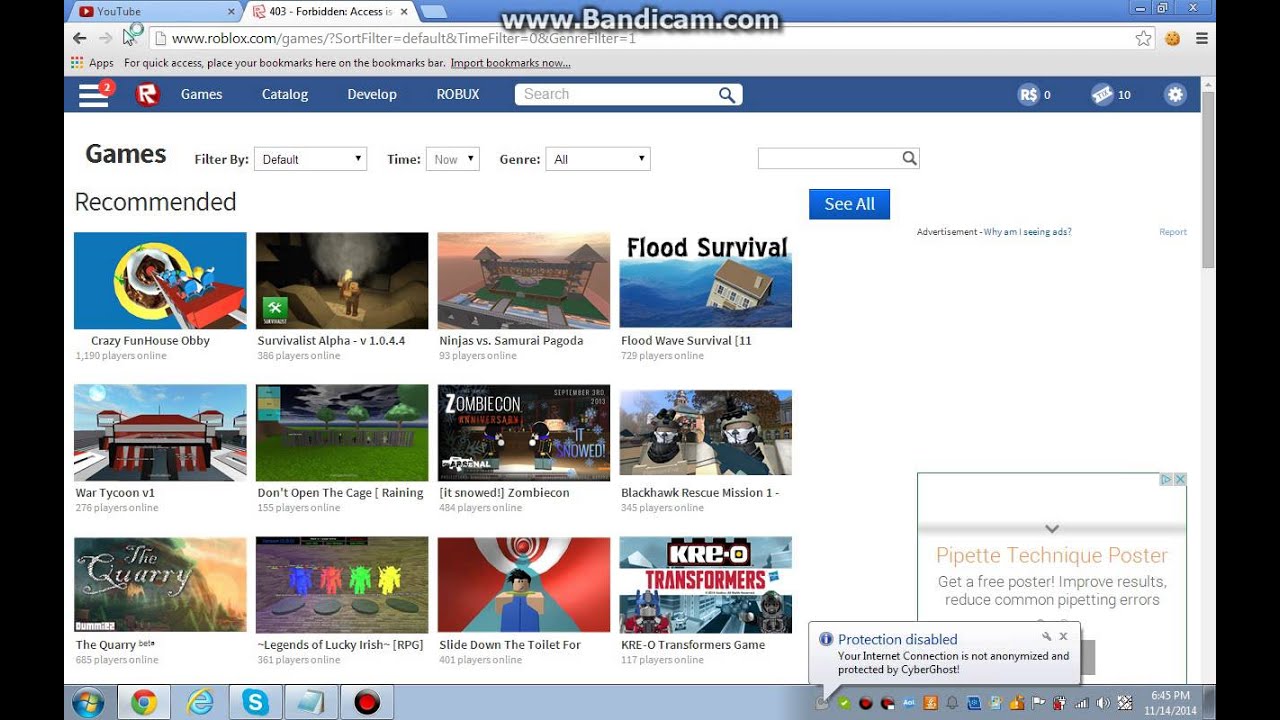This screenshot, evidently captured from a desktop computer, displays two open tabs within a web browser, framed by vertical black bars on either side. A watermark at the top center reads "www.bandicam.com," indicating the use of screen capture software. The left tab is labeled "YouTube," while the right tab, which is in focus, shows a "403 Forbidden" access error message. The URL in the address bar of the active tab is "www.roblox.com/games/?sortFilter=default&timeFilter=-Q&genreFilter=-1." Below the address bar, a purple navigation banner features white text that reads "Games Catalog Develop Robux," alongside a white search field with a purple magnifying glass icon.